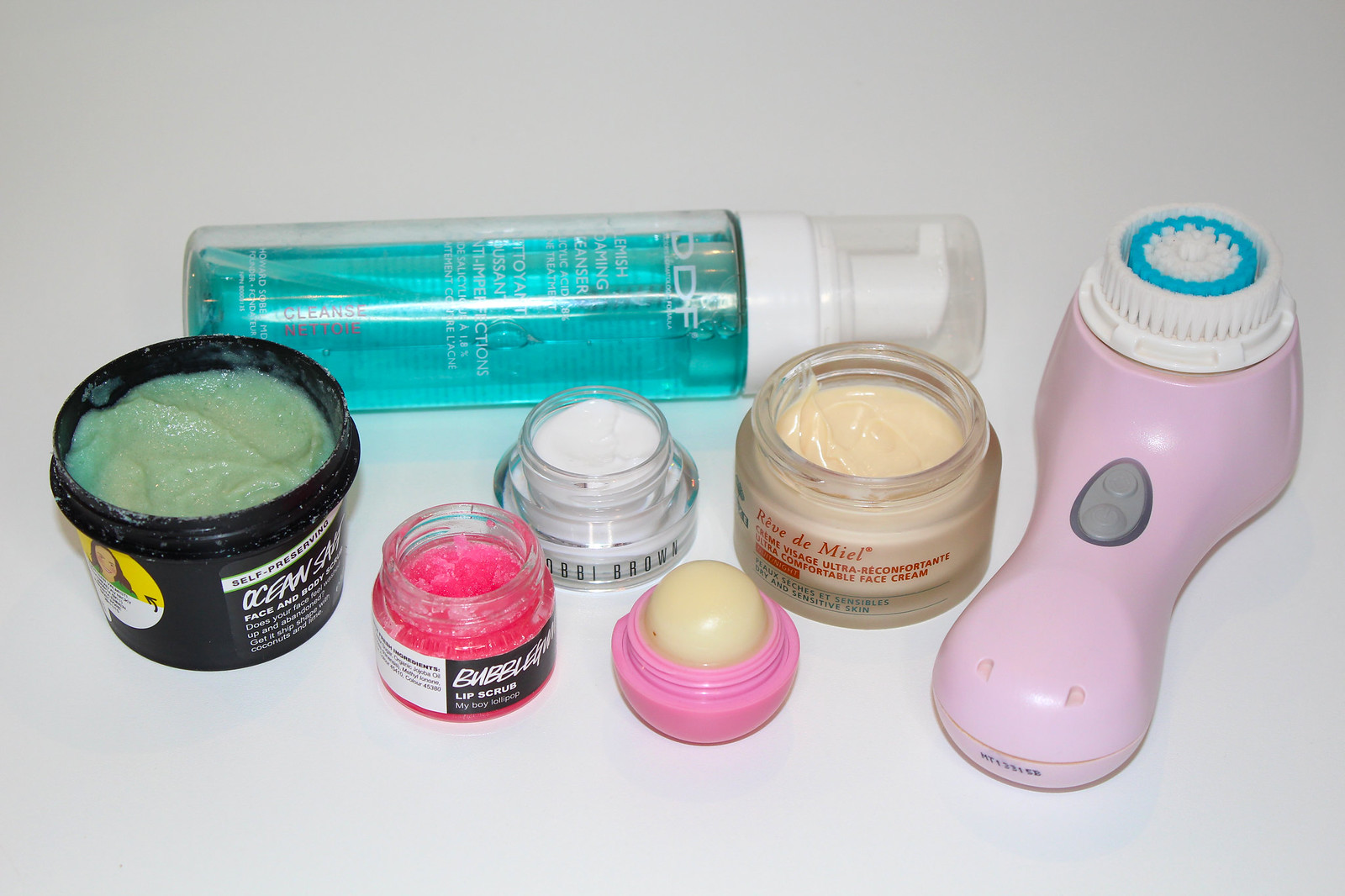A meticulously arranged collection of skincare products is displayed in the photograph, consisting of six distinct items and one tool specifically designed for facial care. Central to the composition is a pink, hourglass-shaped face scrubber, featuring a white and teal concentric brush head and a gray on/off switch with a trigger position.

To the left of the face scrubber, an open jar of Reve de Mille Ultra-Comfortable Face Cream reveals its luxurious contents. Adjacent to it, there is an open container of Bobbi Brown cream, its white substance visible. Moving further left and closer to the camera, an open jar labeled "Bubble Gum Lip Scrub" – boasting a playful tagline "My Boy Lollipop" on its base – showcases its light pink, almost red, exfoliating content.

To the right of the face scrubber, an applicator with a beige wax or ball set in a pink holder is seen. On the far left, a larger black jar labeled "Face and Body Scrub" contains green, gritty material. Positioned behind these items and lying on its side is a pump bottle labeled "Cleansnetoy," filled with a blue liquid and capped securely, indicating it is full.

Each product, meticulously detailed, underscores a comprehensive skincare routine, set against a neutral backdrop that emphasizes their varied textures and vibrant colors.